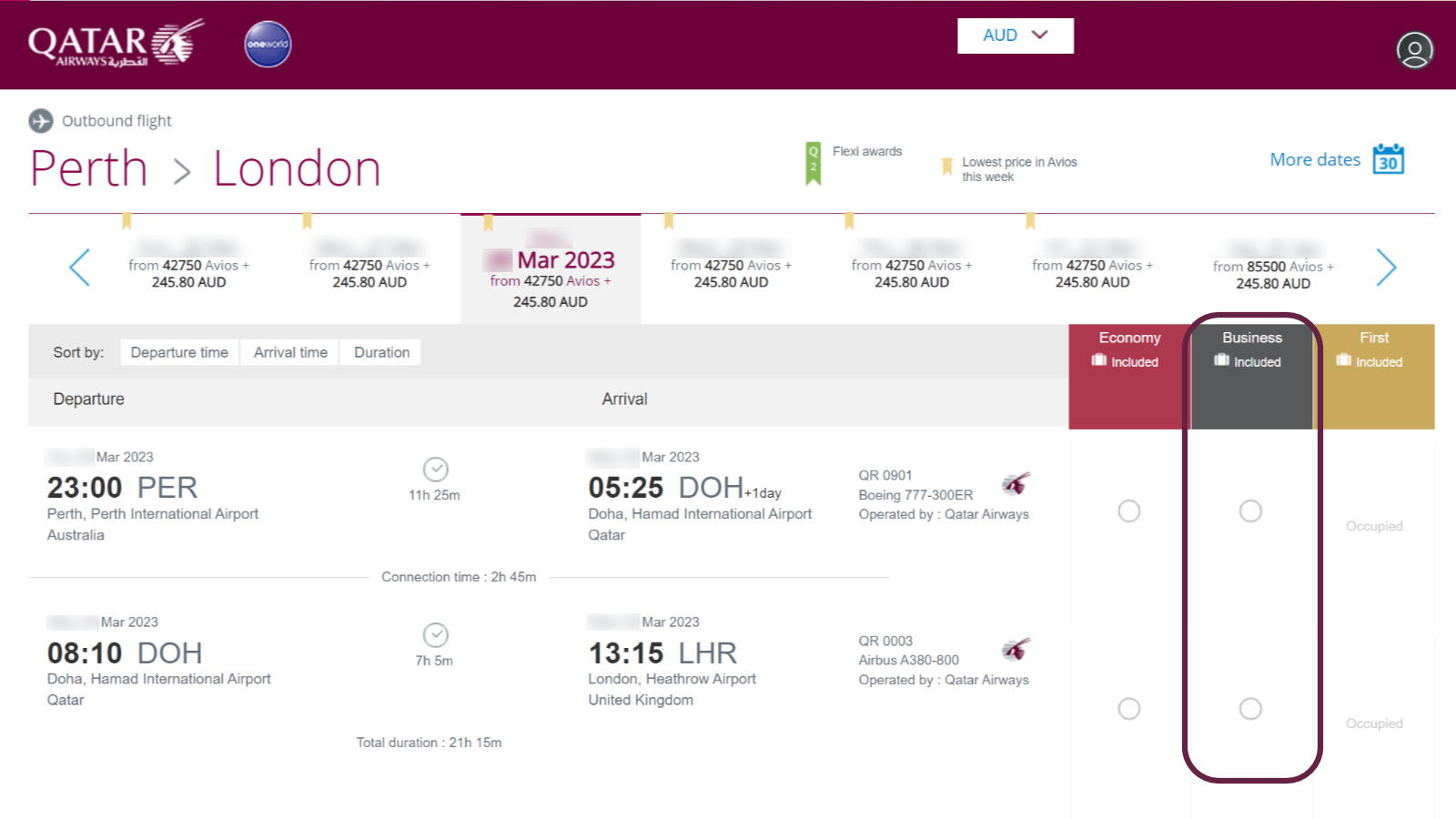Here is a detailed and cleaned-up caption for the described image:

---

This screenshot captures a website displayed on a monitor, showcasing flight information from Perth to London. Dominating the top of the webpage is a burgundy horizontal banner. On the left side of this banner, the word "Qatar" is prominently featured in large, bold, white letters. Adjacent to it is an oval or circular logo with white detailing on its right side. Below the logo, in smaller white text, it reads "Airways," though the font is notably tiny. Further right, there is a blue circle outlined in white, containing illegible white text due to its small size. On the far right of the banner, a small white button for searching or filtering is visible, beside which the currency indicator "AUD" is displayed in blue, accompanied by a maroon-colored downward arrow. Additionally, a grey circle with a white outline features a human icon.

Beneath the burgundy banner, the webpage continues with a white background. Here, the text "Outbound Flight" appears alongside a gray icon of a plane on the left. Above this section, in maroon text, the route "Perth → London" is indicated. Following this heading, various dates and fares are listed, though much of this information is redacted with a smoky gray blur. One visible entry shows, in the center, the fare for March 2023: "From 42750 Avios, $245.80 AUD" written in burgundy text. Additional fare amounts to the right are similarly blurred on the upper lines.

Below this, a gray horizontal banner offers sorting options for the flight details, including "Departure Time," "Arrival Time," and "Duration." This banner is divided into sections with "Departure" on the left, "Arrival" in the center, and three colored squares on the far right: a red square, a gray square, and a mustard-yellow square.

A deep maroon oval highlights the business section column in the center. Below this, two rows of flight times are displayed. The first row indicates a departure time of 23:00 from Perth, arriving at 05:25. The second row shows a departure time of 08:10, with an arrival at 13:15.

---

This caption offers a comprehensive and detailed view of the elements present in the screenshot, providing clear context and descriptions of each part of the webpage.